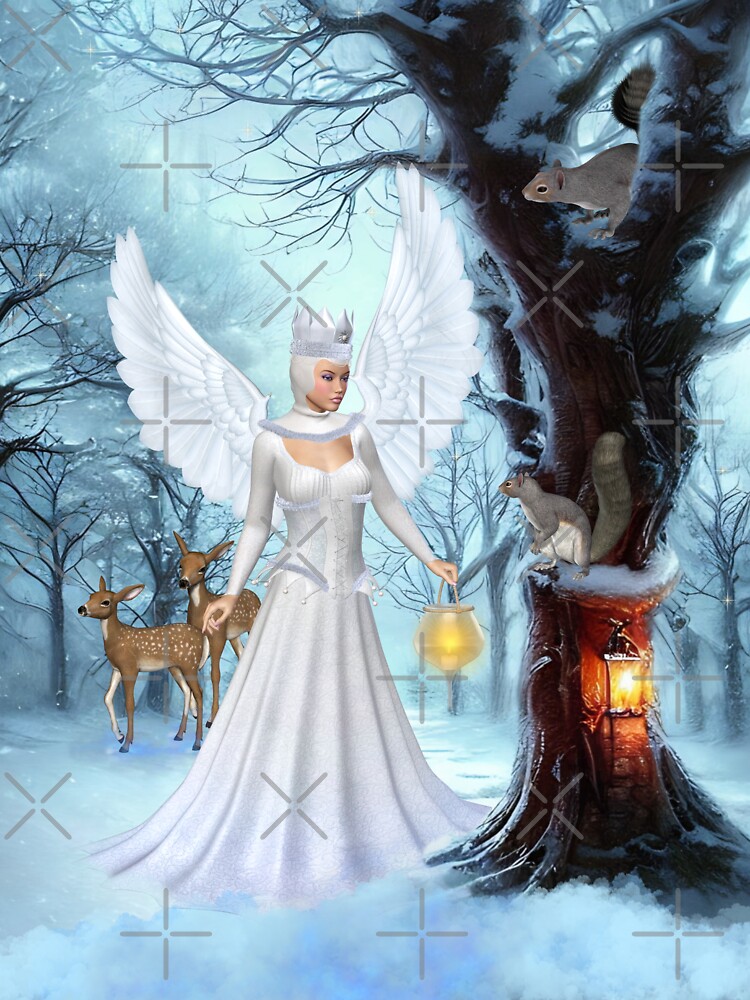This painting portrays a wintertime scene set within a forest, centered around a graceful female angel or perhaps a snow queen. She stands out with her white wings, dress, hair, and crown or halo, holding a lantern in her left hand that casts a soft glow. The angel is gazing at two unusually large squirrels perched on a tree that features a lantern carved into its trunk. To her right, on the left side of the painting, stand two young whitetail deer, brown with white spots, adding to the serene yet whimsical atmosphere. The ground is blanketed with snow, enhancing the wintery ambiance. This image has an early 2000s digital graphic feel, where the distinct elements like the angel, animals, and lantern appear superimposed over a hand-drawn winter forest background. Additionally, sporadic gray crosses and X’s are scattered throughout the painting, possibly serving as a watermark, contributing to the overall low-quality, cartoony feel as though it were rendered by AI.